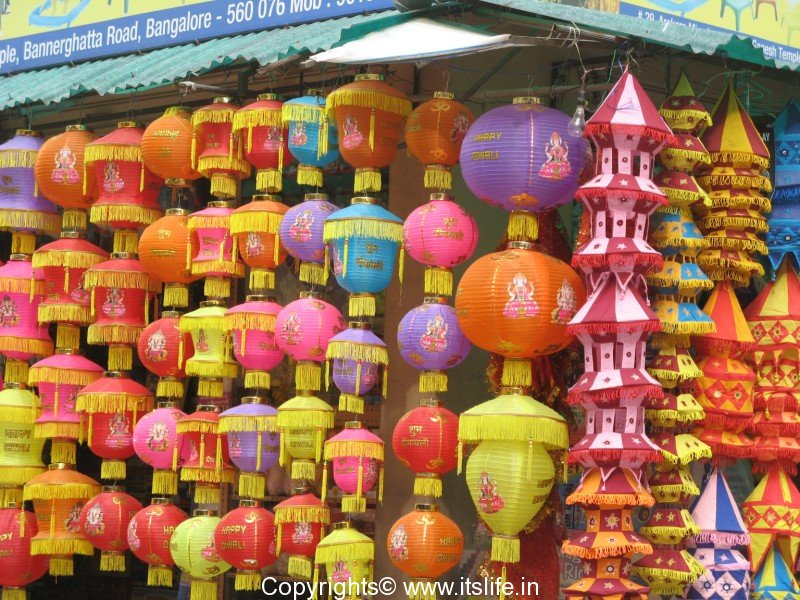The image depicts a vibrant storefront along Banner Gata Road in Bangalore, India. The storefront is completely adorned with an array of colorful lanterns, effectively obscuring the shop itself from view. Above the storefront, a sign reads "Banner Gata Road Bangalore 560-076," though part of the text is cut off. The lanterns, which come in various shapes, colors, and sizes, hang predominantly from a green overhang. Predominantly, the lanterns are spherical with yellow tassels, in hues of orange, pink, purple, yellow, and light blue. Mixed among these are unique designs, including alternating white and red stripes and star patterns. Some lanterns are shaped like pagodas, particularly concentrated on the right third of the scene. The lanterns are of various sizes, ranging from large pumpkin-like forms to smaller, volleyball-sized ones. Additionally, some lanterns have inscriptions such as "Happy Diwali," adding a festive touch. At the bottom of the image, the text "copyright www.itslife.in" is visible, indicating the image’s source. The photograph appears to be of an outdoor market or stall specialized in decorative lighting, capturing the essence of a lively and colorful marketplace in Bangalore.